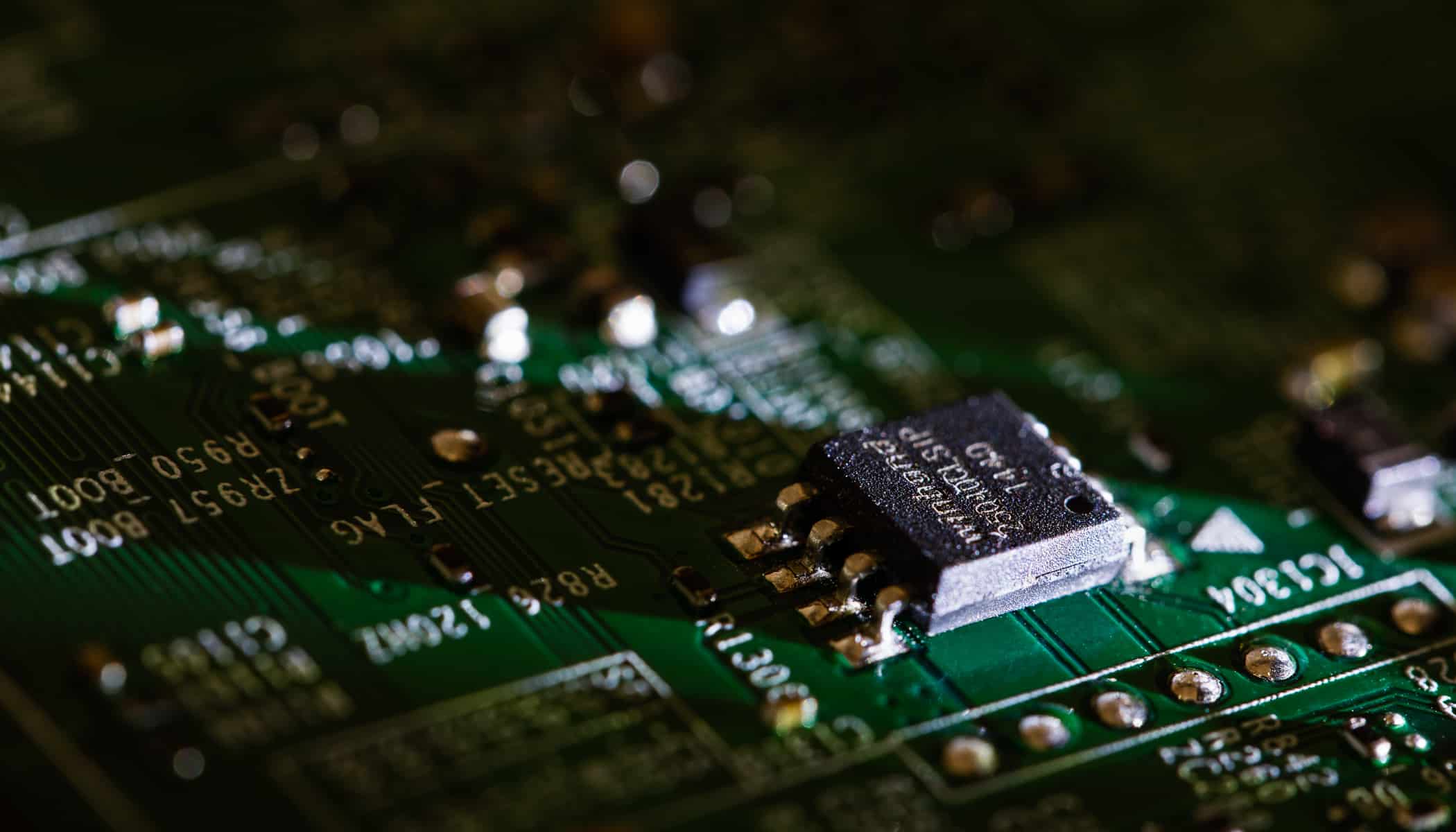This highly detailed, close-up photograph showcases a green printed circuit board (PCB) with a distinct focus on a centrally positioned black microchip. The microchip, which has a white numerical serial number on its surface, is soldered securely into the PCB. Surrounding the microchip, the board is populated with various metallic components and connection nodes, discernible through the white alphanumeric labels, rendered in a clear sans-serif font. Particularly notable are the seven metal circular dots located in a white box at the lower right corner of the image. Above this box is a rectangular shadow, cast by the raised microchip, which extends to the left-middle portion of the frame due to light shining from the right. Among the visible labels on the PCB are "RESET FLAG" and "ZR957N BOOT," although these, along with others, appear upside down, indicating the image's orientation. Despite the extensive array of components, the sharp focus on the black microchip emphasizes its significance in the intricately detailed composition of the circuit board.